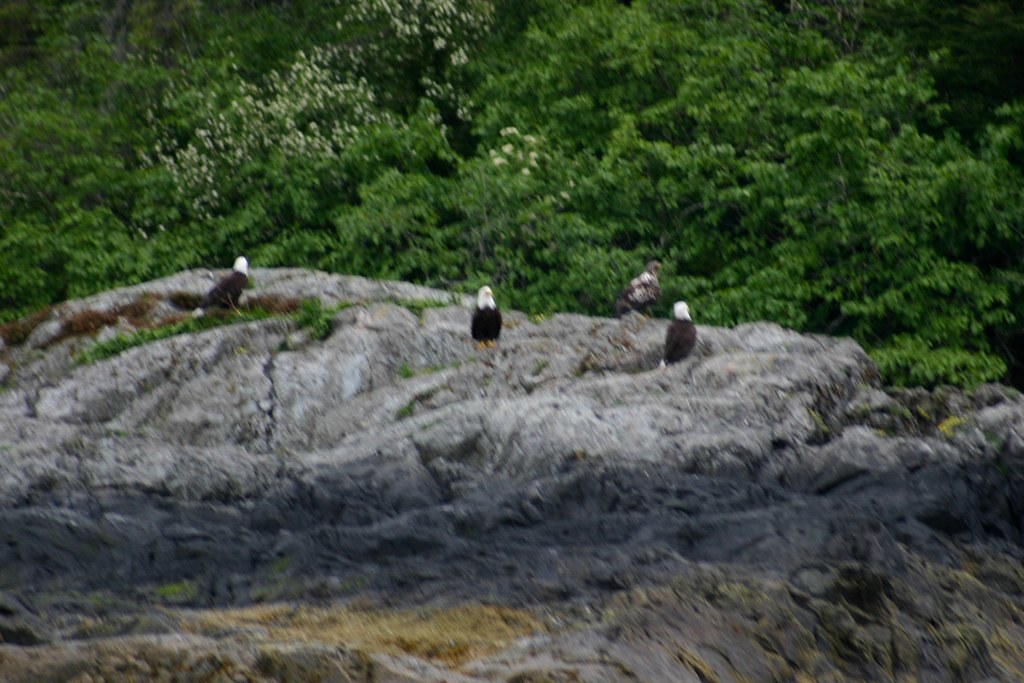The image depicts a striking outdoor scene featuring a large, rugged cliff side, likely the upper part of a mountain with a steep slope visible towards the bottom right. The bare stone face of the cliff is prominent and expansive, marked with a mix of gray and rough brown textures. Perched atop this towering rock formation are three iconic birds with distinctive white heads and dark brown bodies, most probably bald eagles, although the distance and image blur make it challenging to identify them with absolute certainty. Behind this rocky outcrop stretches a dense forest, where a canopy of vibrant green trees is interspersed with several that bear delicate white blossoms, adding a touch of contrast and beauty to the verdant backdrop despite the image's overall lack of sharp detail.